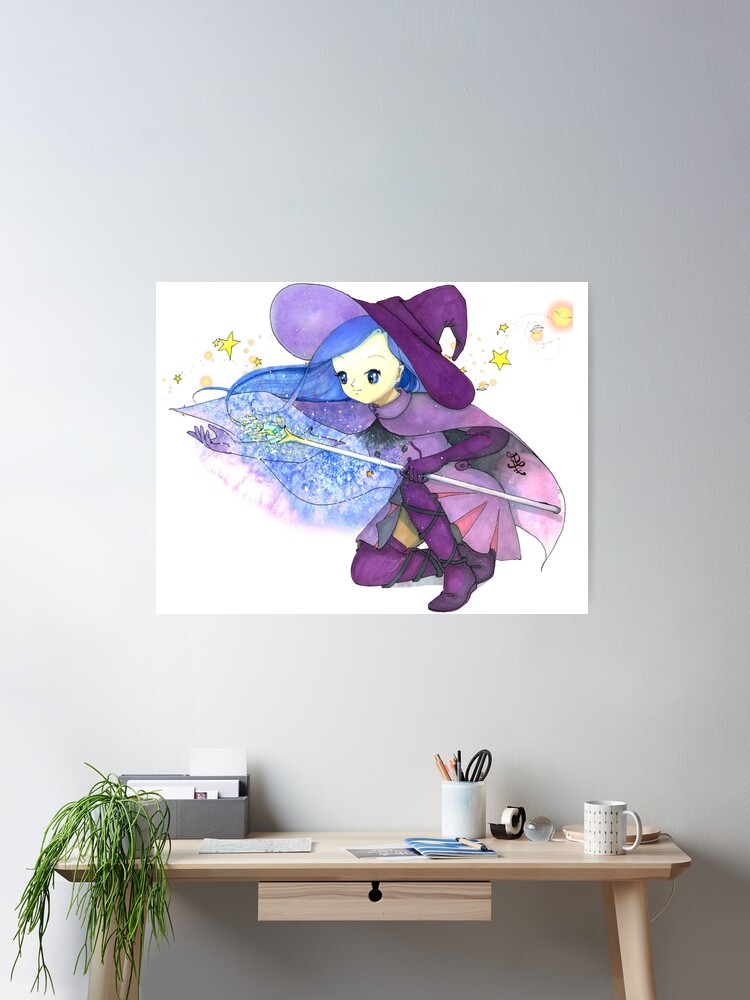This is an indoor photograph featuring a small wooden desk against a very light gray, almost white, wall. The modest desk has slender spindly legs and a thin top with a centrally placed, laptop-sized drawer beneath it. On the desk's surface, there is a coffee cup, a desk lamp with a tubular light, a small plant with dangling foliage on the left side, and a gray box resembling a miniature file cabinet. A cup filled with scissors, pencils, and pens, along with some tape and scattered papers, completes the desk's clutter.

Above the desk, a vibrant poster depicting an anime-like young witch captures attention with its colorful details. The teenage witch, set against a white backdrop, features striking blue hair and large expressive eyes. She dons a big purple witch’s hat with a lighter purple brim, a matching cape, a dress with purple accents, purple boots, and socks that rise above her calves. She is kneeling and appears to be casting a spell, holding a wand with a greenish jewel at its tip, surrounded by scattered yellow stars and a light blue aura. The character’s whimsical design adds a splash of purples, blues, and yellows to the otherwise muted room.